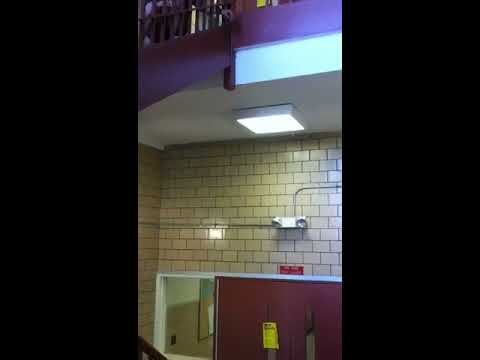The photograph depicts an indoor hallway of a building, likely a school, showcasing several architectural and safety features. Dominating the lower section is a brown door fitted with a small white window, surmounted by a red sign, the text of which is not legible. This sign is affixed to a light-colored, subway-style brick wall. Flanking the doorway are two emergency lights, accompanied by a fluorescent light mounted on the white ceiling above. The ceiling's white appearance subtly transitions to a purplish hue in some areas due to the lighting. Further up, a window reveals a dimly lit, grayish-blue exterior. Adjacent to the main visual components are some silver fixtures and what appears to be stairs behind the door—hinting at an entryway or an emergency exit leading to an upper floor. Lighting from the ceiling casts a noticeable glow over the scene, enhancing the overall visibility and emphasizing the structured layout of the hallway.